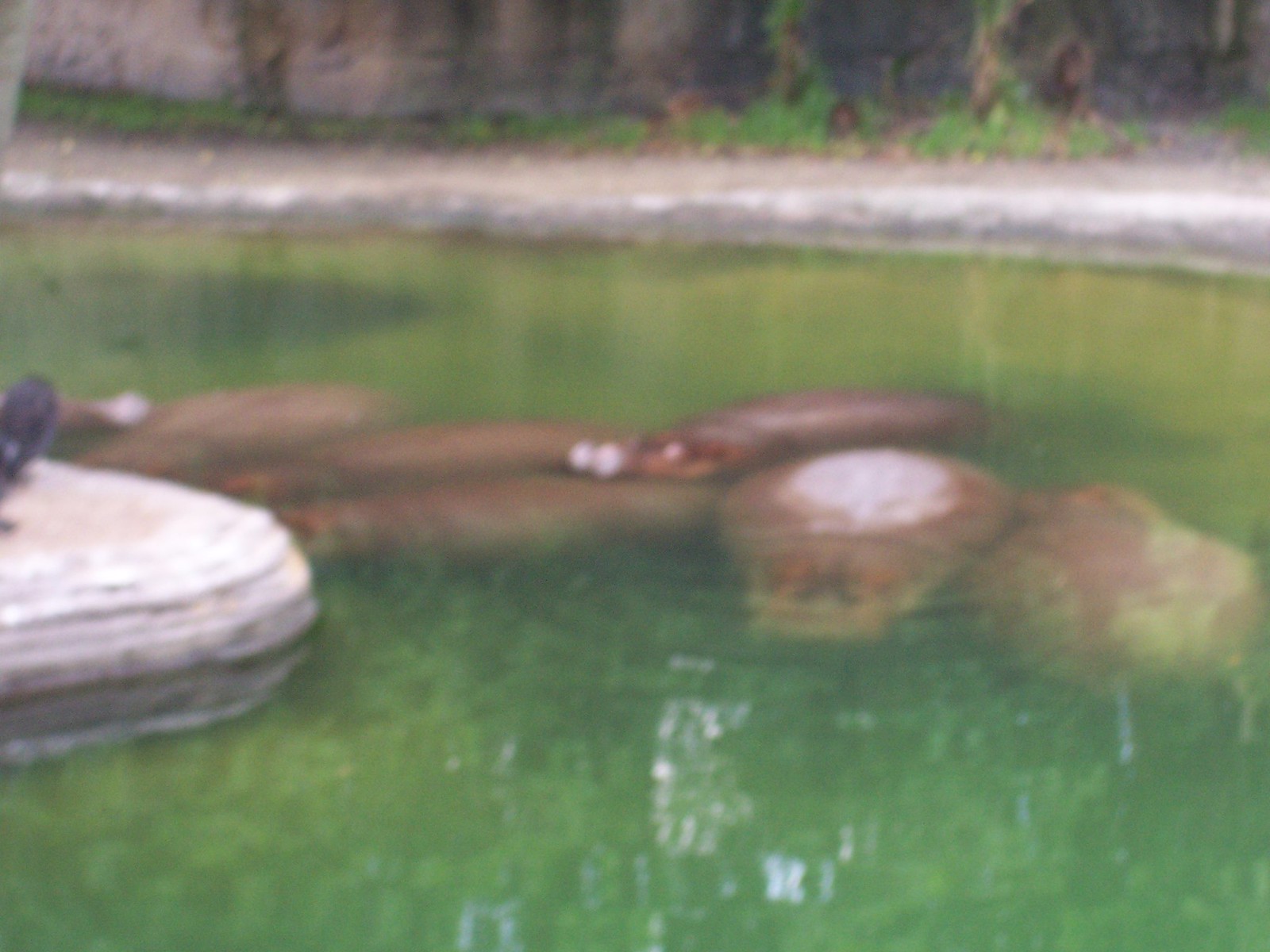This impressionistic and extremely blurry photograph captures a serene, green-hued body of water that stretches almost to the top of the image. In the foreground, large, rounded, and oval-shaped rocks are partially submerged, with their gray tops peaking out just above the dark brown waterline. Among these rocks, one appears to have a turtle resting on it, while another observer mentions a black bird standing on a rock or a peninsula-like feature. There is a suggestion of several manatees horizontally stretching across the photo, with one slightly breaking the water surface. The water itself is green and hazy, indicating the presence of algae, and strands of what may be grass float near the bottom. Along the top edge of the image is a narrow strip of land adorned with sparse greenery and brown tree trunks, with the land possibly rising to form a hill or a cliff. The photograph, though pixelated and extremely blurred, conveys a tranquil natural setting.